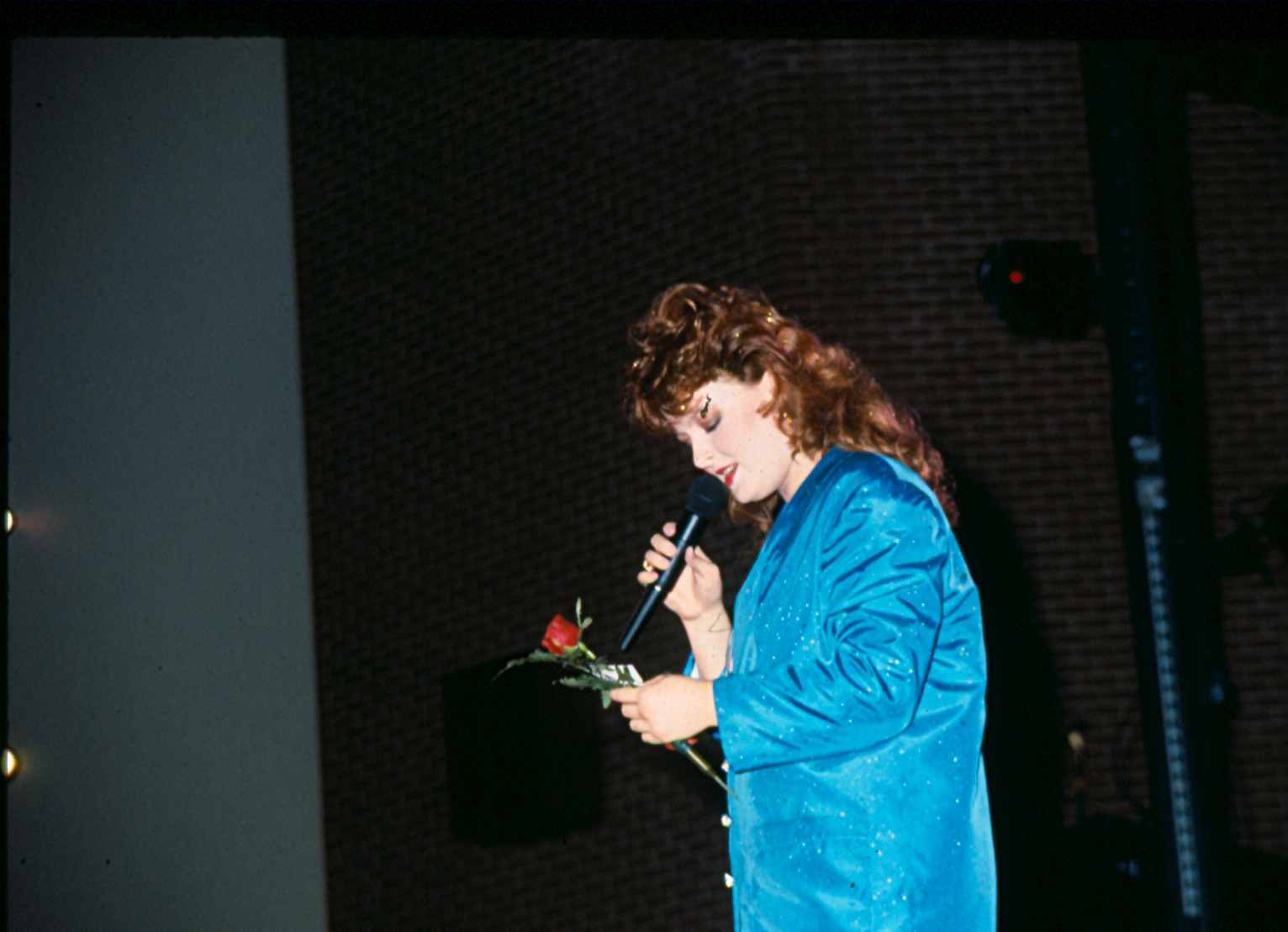This is a photograph of Weona Judd, captured in an interior setting that features a tall brick wall and lights along a white surface to the left, suggesting an auditorium stage. Judd, a white woman with long, curly reddish-auburn hair flowing past her shoulders, exudes glamour with her meticulous makeup that includes red lipstick and eye shadow. She is dressed in a shiny, possibly sequined, blue satin jacket which sparkles under the stage lights. In her left hand, she holds a red-petaled rose with a green stem along with a white note card, at which she is intently looking down. Her right hand grips a black microphone held to her lips as she speaks. The overall atmosphere of the image hints at a performance from the 1980s, portraying Judd's engaging presence on stage.